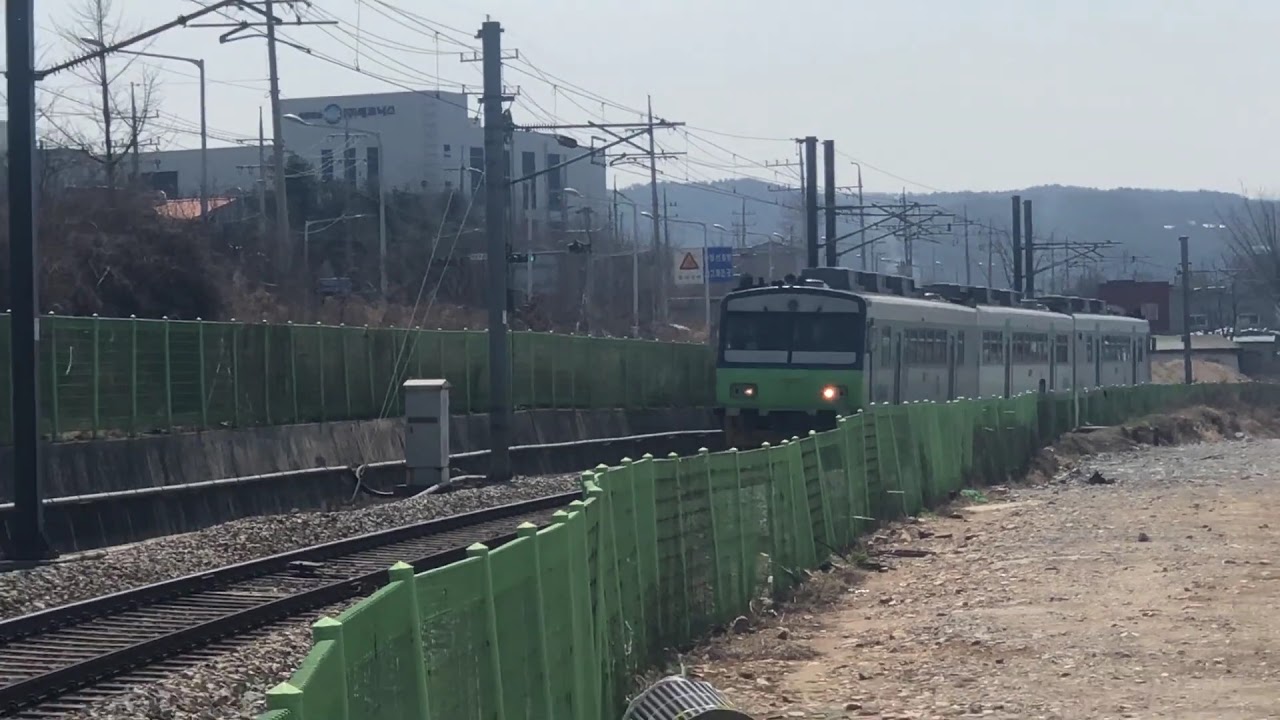The photograph captures a green and gray light rail train traveling through an industrial and somewhat underdeveloped part of town. The train, composed of three cars with visible yellow headlights, runs along tracks bordered by a green plastic or metal fence that matches the train's color. To the right of the train, the scene features barren dirt, resembling a neglected or vacant area, possibly a construction dump-off point. On the left, there are numerous tall posts supporting an intricate web of power and telephone lines, adding to the industrial atmosphere. Behind these posts, we can see factory-style housing and a white building. The sky appears overcast, enhancing the gritty character of the location. A sign in the distance hints at a gas station, though it's hard to discern its specifics. This area, separated from more populated city sections by the green fence, underscores the stark contrast between the developed and undeveloped parts of the city.